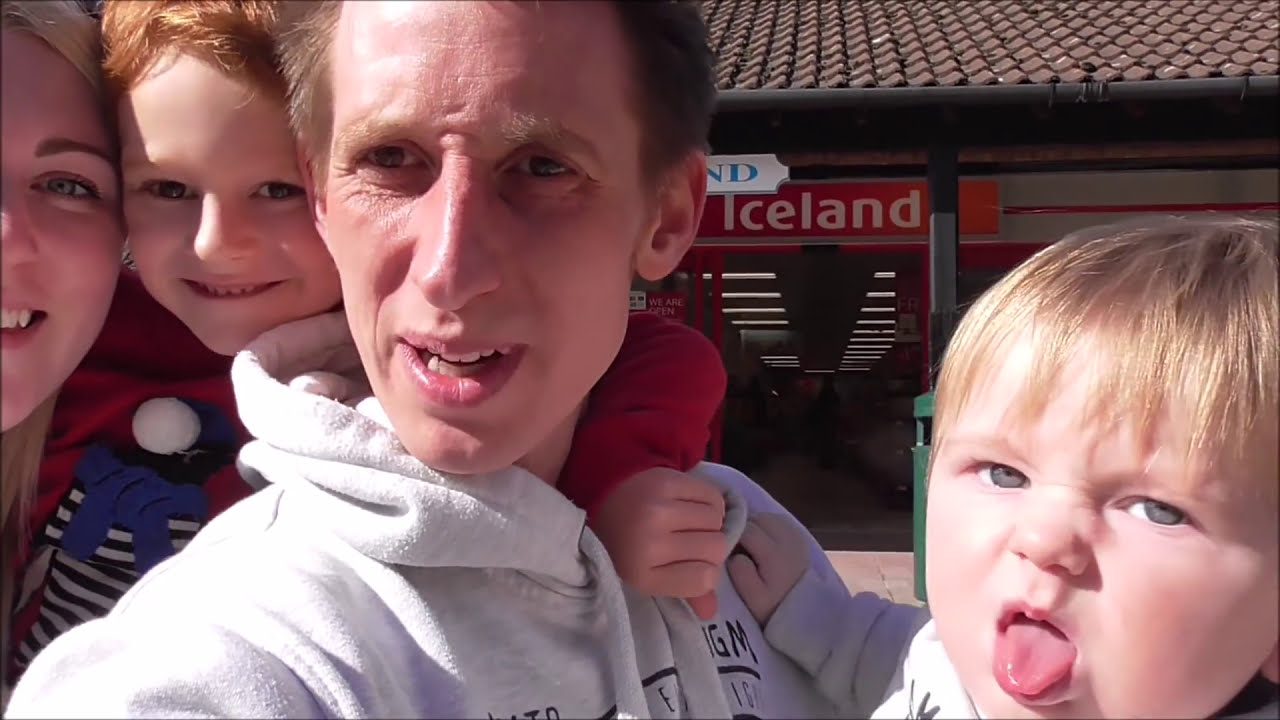This is a detailed selfie of a family of four, taken in front of a store called Iceland. The main subject, likely the father, is in the center wearing a white hoodie jacket. He has a serious expression and is probably in his forties. To his right, he holds a small blond toddler, likely a boy, who is sticking out his tongue at the camera. To the father's left, a red-haired child with brown eyes, who appears to be around three or four years old, is smiling warmly. In the far left, the partial face of a woman, likely the mother, with blond hair, is visible, and she is also smiling. The backdrop features a building with brown roof tiles and a sign that reads "Iceland," suggesting the family might be at or near a travel station about to embark on a journey. The selfie captures their upper bodies and faces vividly against this background.